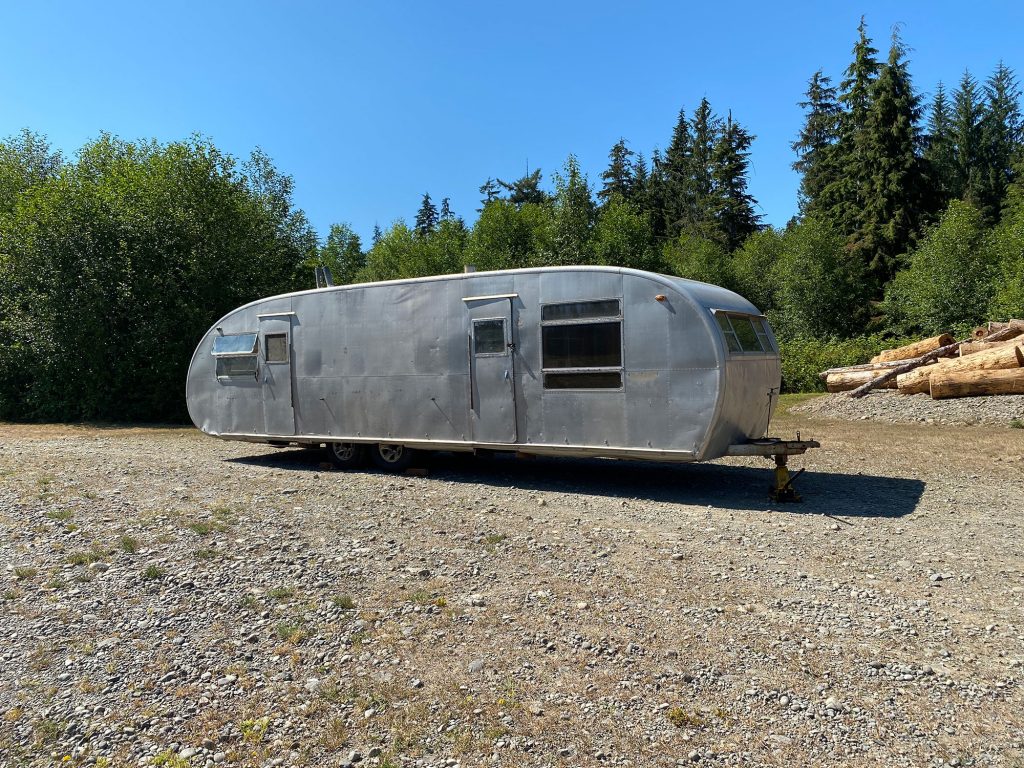The image depicts an antique, silver-colored camp trailer with a rounded shape parked on a gravel surface under a clear blue sky. The trailer, which is quite long, casts a shadow to the right. It features two doors, each with a central window, and multiple sets of windows. On the right side at the front, there's a large central window flanked by narrower ones on the top and bottom. The rear window is divided into two sections, with the upper section slightly open. At the front of the trailer, there is another set of windows with a main window in the center and smaller sections on either side. The hitch at the front of the trailer extends outwards and casts a substantial shadow to the left. Surrounding the trailer are tall, green pine trees to the right and dense, leafy trees to the left. Additionally, there is a pile of smooth, cut-up logs on the right side.